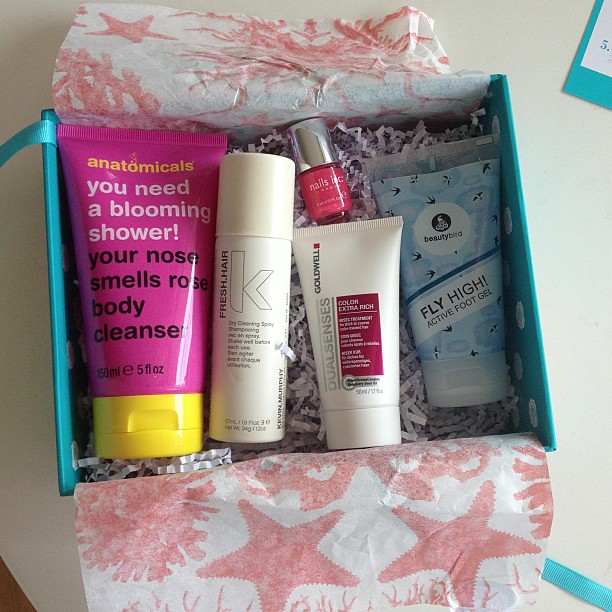This is a professionally-taken photograph of a teal blue beauty care package, elegantly presented on a white surface. The open box reveals a meticulously arranged collection of beauty products nestled in white crinkly packing paper, complemented by tissue paper adorned with pink starfish, plankton, and algae motifs, adding an oceanic theme to the presentation. Visible in the background are hints of blue, possibly from a page or ribbon, enhancing the cohesive color scheme.

The contents include:
1. A large pink tube with a yellow cap labeled "Anatomicals". The branding on it reads, "You Need a Blooming Shower! Your Nose Smells Rose Body Cleanse," containing 5 fluid ounces.
2. A white tube with a red square titled "Color Extra Rich," part of the DualSenses line by Goldwell.
3. Another white tube, vertically inscribed with "Fresh.Hair" by Kevin Murphy, likely a dry shampoo, detailing "Dry Cleaning Spray Shampooing" and advising to "Shake Well Before Each Use."
4. A small bottle of "Nails Inc" nail polish with a silver lid, displaying a pink hue.
5. Lastly, a blue, black, and white tube tagged "Beauty Bird Fly High Active Foot Gel."

A partially visible envelope marked with the number 'five' is placed nearby, adding a touch of mystery to the gift set. The curated assortment of products suggests it could be a subscription beauty box, meticulously designed to delight any recipient.